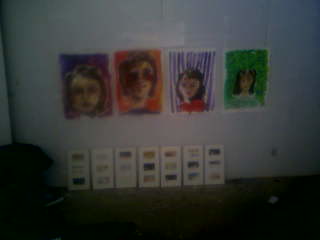The image is a small digital photograph depicting a dimly lit, shadowy room with an unsettling ambiance. The focus of the image is a white wall adorned with four rectangular portraits, seemingly drawn with crayon, possibly by children. These portraits depict Caucasian women with varying backgrounds: 

1. The first portrait on the left has a pink or purple background with a woman who has light brown hair. The facial features are indistinct.
2. The second portrait features an older woman with yellowish hair against a greenish background, her eyes appearing black.
3. The third painting shows a woman with dark brown hair and a pink shirt set against a circularly patterned, purple and white background; the facial details are virtually unrecognizable.
4. The fourth portrait, under a green background, depicts a younger woman with a center-parted dark brown hair and a light green shirt.

Below these, leaning against the wall, are either seven or eight smaller triangular pieces containing several tiny rectangles of different colors, though their details remain unclear due to the dim lighting and low resolution.

The lower portion of the image reveals more context: a nasty, dirty brown carpet and a beanbag chair, nearly black, are visible on the floor. The presence of a wall outlet is also noted but doesn't add significant detail to the primary focus. The overall dark and shadowy quality of the image contributes to a creepy, almost eerie feeling.